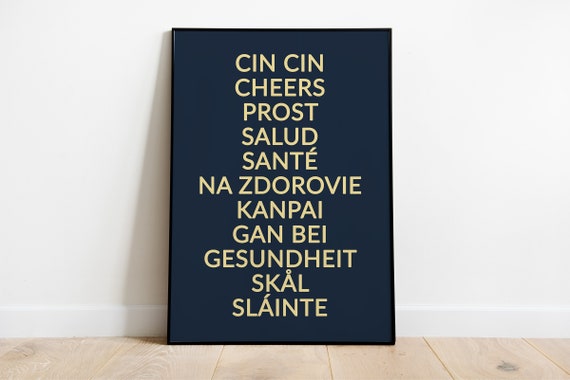The image showcases a rectangular, framed poster in a minimalist setting, ideal for product display. The poster is encased in a thin black frame and is positioned horizontally, leaning against a crisp white wall. The floor beneath it features light brown, almost blonde, wooden planks. The poster itself has a deep navy blue background, highlighted by bone white or yellowish light text. This stylish piece of decor lists various ways to say "cheers" in different languages, making it perfect for a bar or man cave. Prominently featured from top to bottom are the words: Cin Cin, Cheers, Prost, Salud, Santé, Nâzdar, Zdorovye, Kanpai, Gambai, Gesundheit, Skål, and Sláinte.